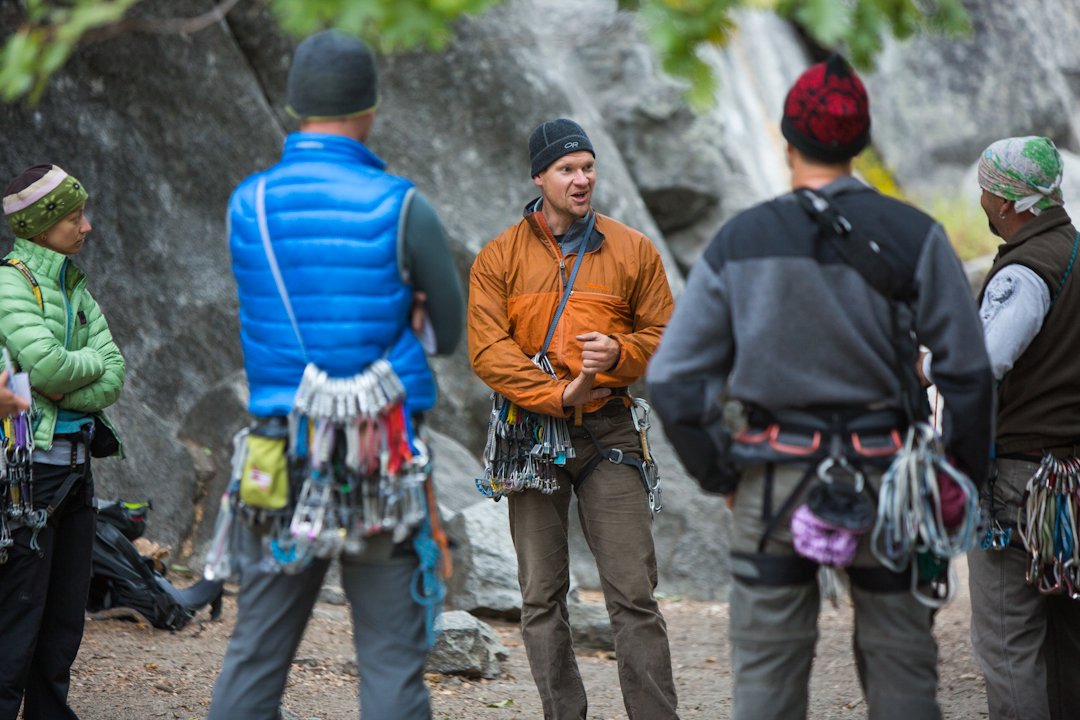The image captures a group of five people, clearly preparing for a rock climbing adventure amidst a scenic backdrop of rocks and a waterfall. Central to the composition is a man in an orange coat and brown pants, who stands out as he faces the camera, seemingly engaged in conversation with the group. His hands are clasped, and he wears a knit hat, making him the focal point. Surrounding him, the other individuals, four of whom are also wearing knit hats except for one sporting a white and green bandana, attentively listen. On the left, a woman in a green puffer coat maintains a serious expression with her arms crossed. Next to her is a man in a blue puffer coat, followed by another in a gray, soft-textured shirt. To the right is a man in a brown vest over a white shirt. Notably, all are equipped with numerous carabiners and climbing gear, which underscores their preparedness and experience. The earthy terrain underfoot and the rugged, mountainous setting add to the adventurous atmosphere of the scene.